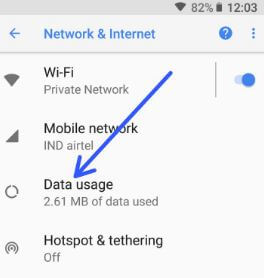The image displays the settings page of a mobile phone, focused on network and internet configurations. At the top of the page, there is a gray status bar showing the Wi-Fi signal, battery level at 82%, battery icon, and the current time of 12:03. Below the status bar, a header labeled "Network & Internet" is present with a circular button and three vertically aligned dots on the right side, and a back arrow on the far left.

The main content of the page features four options presented in a vertical list. The topmost option is "Wi-Fi," which is highlighted in bold. Below it, text reads "Private network." To the left of the "Wi-Fi" label, there is a Wi-Fi symbol, and to the right, a vertical separator and an on/off toggle switch.

The second option is "Mobile Network," also in bold text, with "IND Airtel" written underneath. A triangular icon is positioned to the left of this text. Below this, there is a third entry showing "Data Usage: 2.61 MB" with a circular icon to the left.

The final option at the bottom is "Hotspot & Tethering," with the text "Off" written below it. To the left of this label is an icon representing this function.

Each element is clearly delineated, providing a comprehensive overview of the network and internet settings on the mobile device.